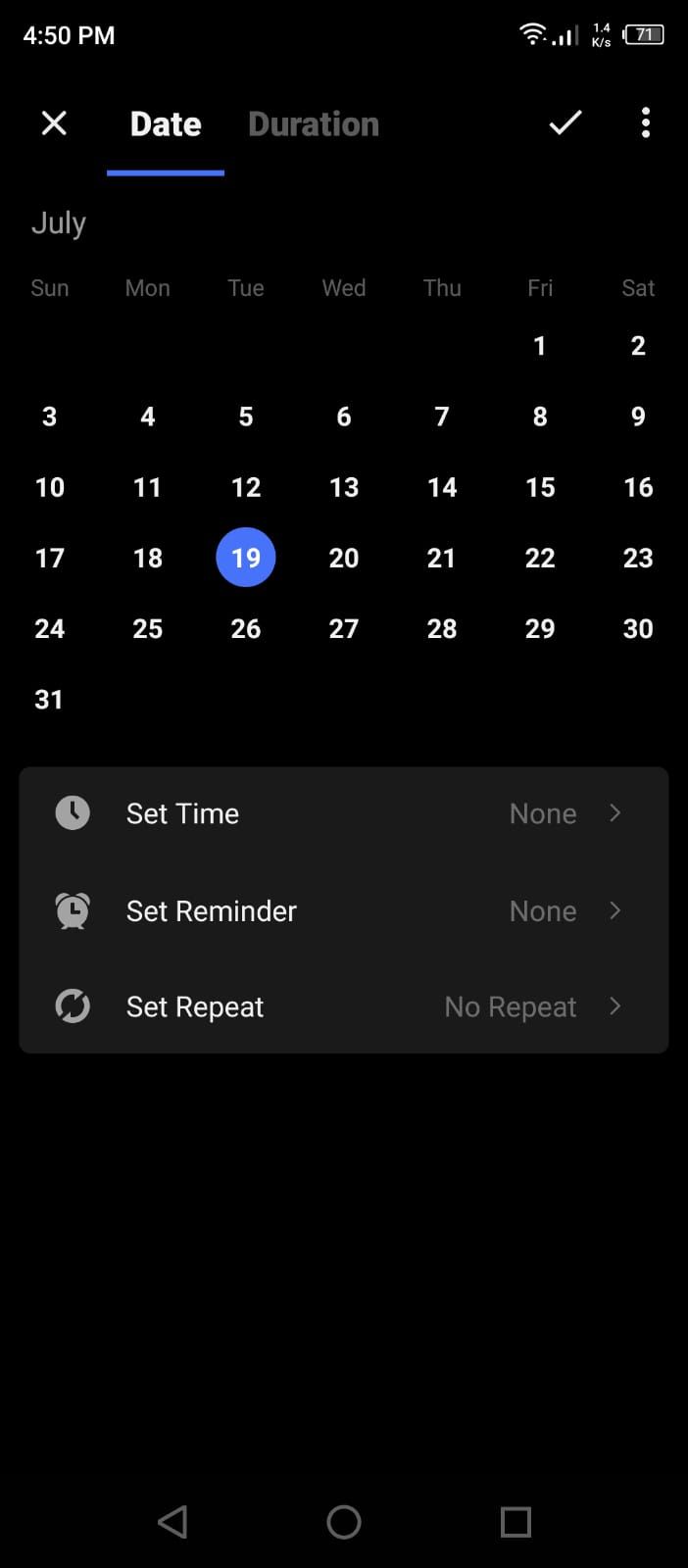A detailed screenshot of a calendar interface showcasing the setup process for an appointment or reminder. The interface features a predominantly black background with white text, providing clear contrast for easy readability. The month displayed is July, with the date "19th" prominently highlighted in blue, possibly indicating the selected day.

At the top of the interface, there is an option to toggle between setting the "date" and "duration," giving users the flexibility to schedule their reminders or appointments with precision. To the right, a check mark and a three-dot menu icon are visible, likely for saving the settings and accessing additional options, respectively.

Further down, the interface presents options for "Set Time," "Set Reminder," and "Set Repeat," each accompanied by the text "none" or "no repeat" and a right-facing arrow to signify that these fields can be customized. This indicates that the user has not yet configured these settings.

Once all the desired settings have been adjusted, the user can finalize the process by clicking the check mark at the top of the screen, thereby saving the appointment or reminder.